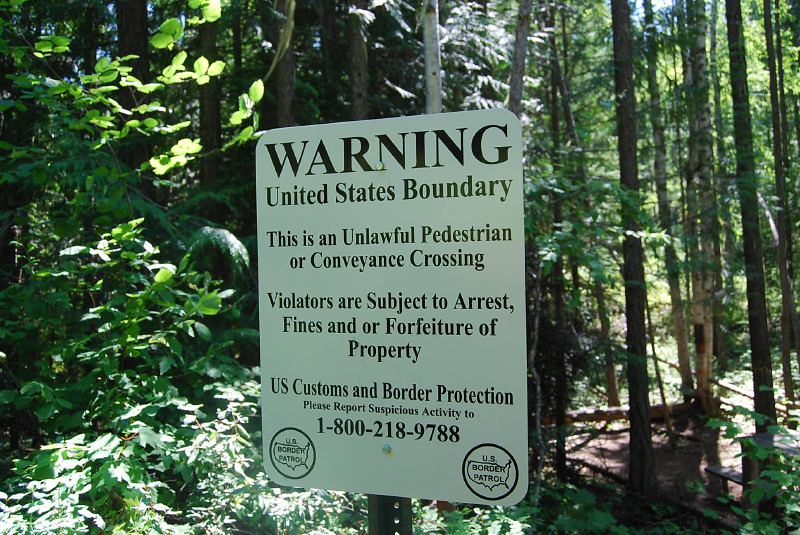This image captures a warning sign prominently displayed in a dense forest. The forest scene is vibrant with lush green trees and bushes, and sunlight filters through the leaves, illuminating the area. The sign itself is mounted on a steel pole and has rounded corners. It bears a stern message in black and white: "Warning, United States boundary. This is an unlawful pedestrian or conveyance crossing. Violators are subject to arrest, fines, and or forfeiture of property." Below this, it is stated, "U.S. Customs and Border Protection, please report suspicious activity to 1-800-218-9788." In the bottom corners, identical logos feature the outline of the United States inside a circle with the text "U.S. Border Patrol." This setting suggests the image is taken at a border crossing area deep within a forested region, capturing the tension between the natural beauty of the woods and the strict border enforcement.